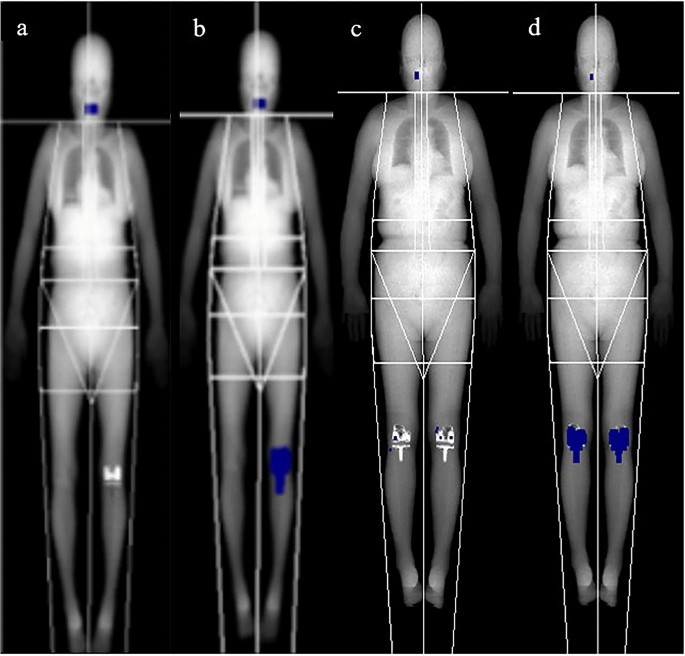This image showcases a four-panel medical scan resembling x-ray imaging, set against a black background with white labels A, B, C, and D from left to right. Each panel contains a full-body scan of different figures, depicted in gray tones. Every figure has blue tape over the mouth area, with additional colored markings on their knees: Panel A features a white mark on the left knee, Panel B displays a blue patch on the left knee, Panel C exhibits white icons on both knees, and Panel D shows blue pieces on both knees. Notably, these images are outlined by white lines that trace the body contours and intersect key areas, including across the neckline, along the body's outline, across the waist, forming a V at the crotch, and extending down the middle of the legs. The figures on the left, A and B, are slightly smaller than the two on the right, C and D, with Panel C being the tallest and slightly broader.